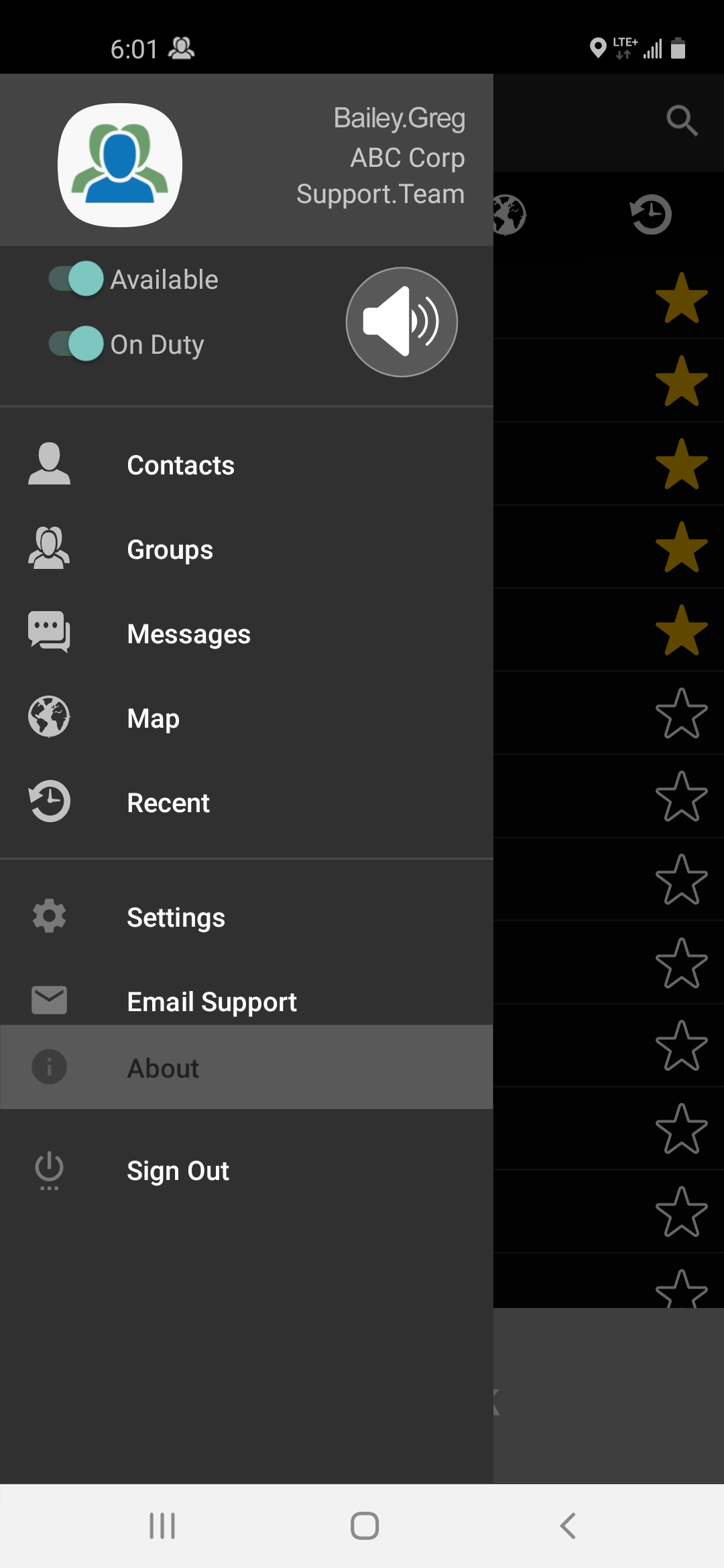Captured on a cell phone, this image depicts a screen with a black background dominated by various on-screen elements and icons. At the top, the status bar displays the time (6:01), network logo, battery icon, and location logo. The main screen shows an app with a side menu that has been clicked open. This menu features a grey bar at the top with an icon of three human faces: the front one is blue, and the two in the background are green, all set against a white background. Beneath this icon, the text "Bailey Gregg ABC Cup Support / Team" appears in grey ink.

Two toggles labeled "Available" and "On Duty" are both switched on, indicated by their blue color. Below these toggles, a sound icon is present, followed by several menu options: Contacts, Groups, Messages, Maps, Recent, Settings, and Email Support, all written in a white or light grey color. At the bottom of the menu, the word "About" is highlighted on a light grey band, written in dark grey or black ink, followed by a "Sign Out" button in white ink.

The background of the screen also features an array of stars. The first five stars are orange, while the remaining stars have a white outline but are not filled in. This adds a distinctive, starry pattern over the predominantly dark background.